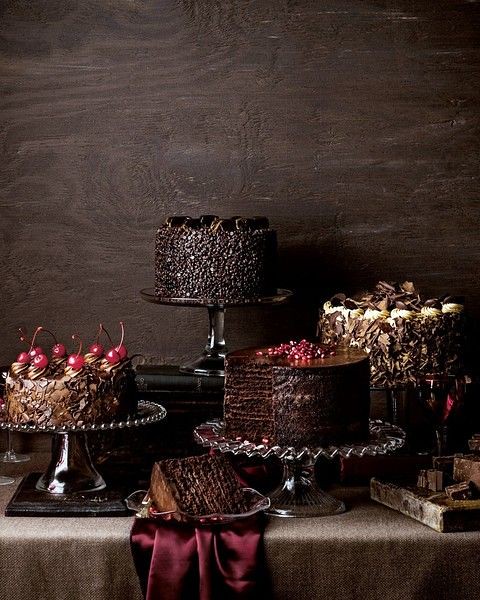This color photograph captures an elaborate display of various cakes arranged on a table adorned with a rich brown tablecloth. The backdrop is a dark wooden wall, its deep chocolate-like wood grain echoing the sumptuousness of the cakes. On the left, an elegant cake stand holds a lighter chocolate cake crowned with a circle of cherries. In the center, a darker, decadent chocolate cake takes prominence, its textured top embellished with chocolate pieces. A single slice of this cake rests below on a plate, set atop a silky burgundy cloth that drapes over the edge of the table. Next to the slice is another cake, missing a piece, revealing a lush red filling and keeping with its chocolate theme. Further to the right, there's a slightly lighter chocolate cake adorned with a ring of white icing near its edge, suggesting a blend of flavors. All the cakes stand at differing heights on dark metallic and crystal cake stands, creating a visually dynamic and lavish dessert display. Just beneath the rightmost cake, a shallow grey wooden box adds an intriguing, though hard-to-distinguish, element to this sweet tableau.